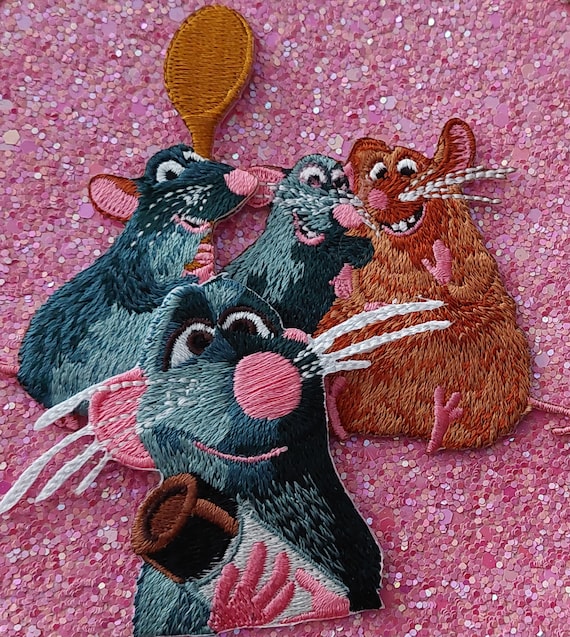The close-up image showcases two embroidered patches, intricately designed with characters from the Disney movie Ratatouille, against a background covered in matte pink glitter of varying sizes and shades. The foreground patch features Remy, the main rat character, who appears proud and happy while holding a small vial. The patch behind him displays three other rats; two look similar to Remy with a grayish-black hue, and the larger, brown rat is distinguishable, possibly holding a wooden spoon. All four rats exhibit expressions of happiness and excitement. The patches, adorned with detailed stitching including whiskers, suggest they can be ironed onto clothing or other fabric materials, creating a delightful and whimsical addition to any garment.